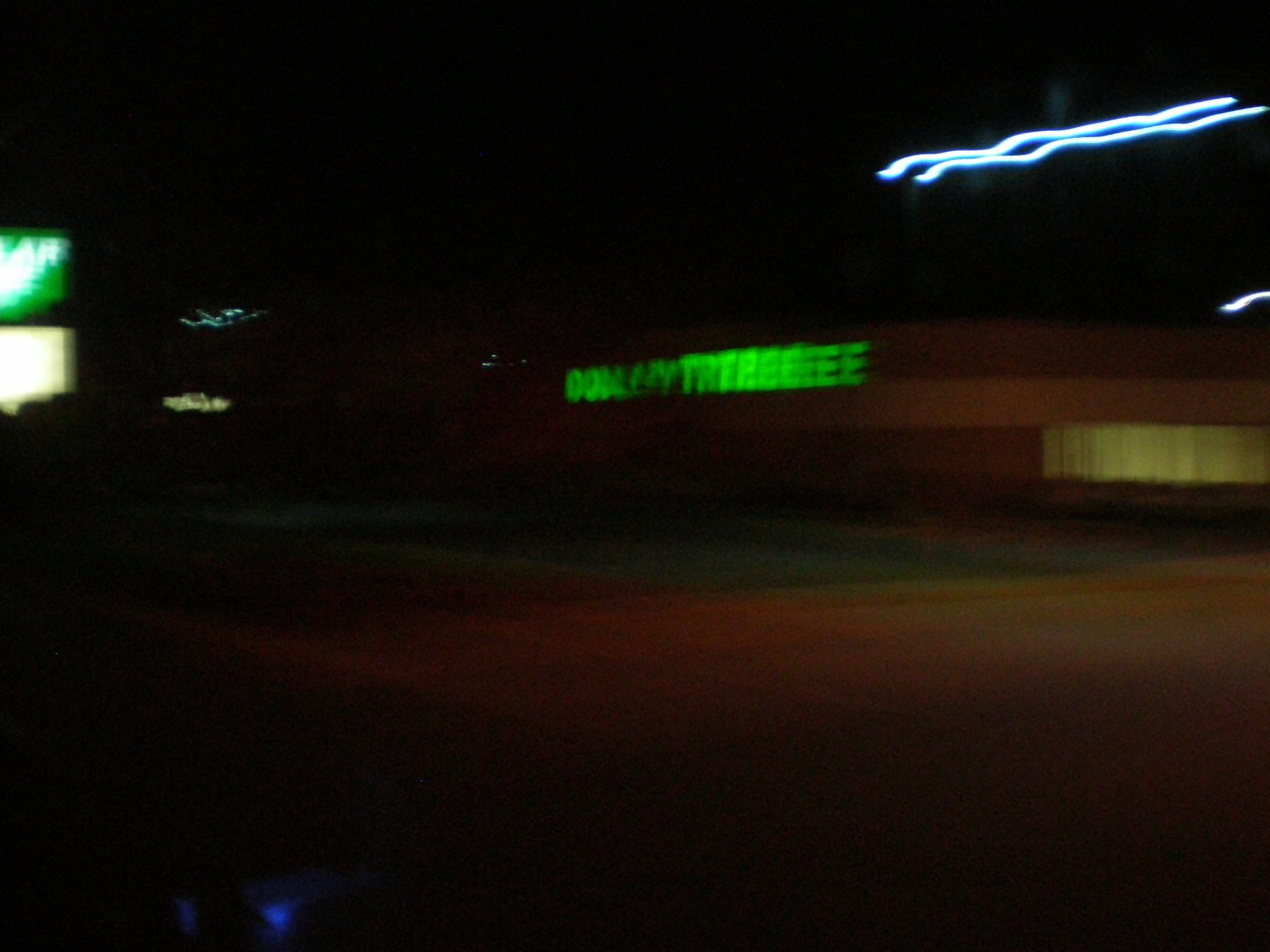The photo is a nighttime shot taken from inside a moving vehicle, resulting in a very blurry and overexposed image. The majority of the frame is shrouded in darkness with a few light reflections appearing as squiggly lines. At the center of the image stands a Dollar Tree store, its large illuminated green sign prominently displaying the name despite being blurred and duplicated due to the motion. The store is situated in a brownish building. Surrounding the store, there are other light sources, including a nearby billboard for the plaza area which features a mixture of blue and yellow lights on the left side. In the top right corner, two bright, neon-like blue lines streak across the image, adding to the out-of-focus effect. Details such as the gray concrete parking lot and windows on the right side of the building are faintly visible against the dark canvas of the photo.